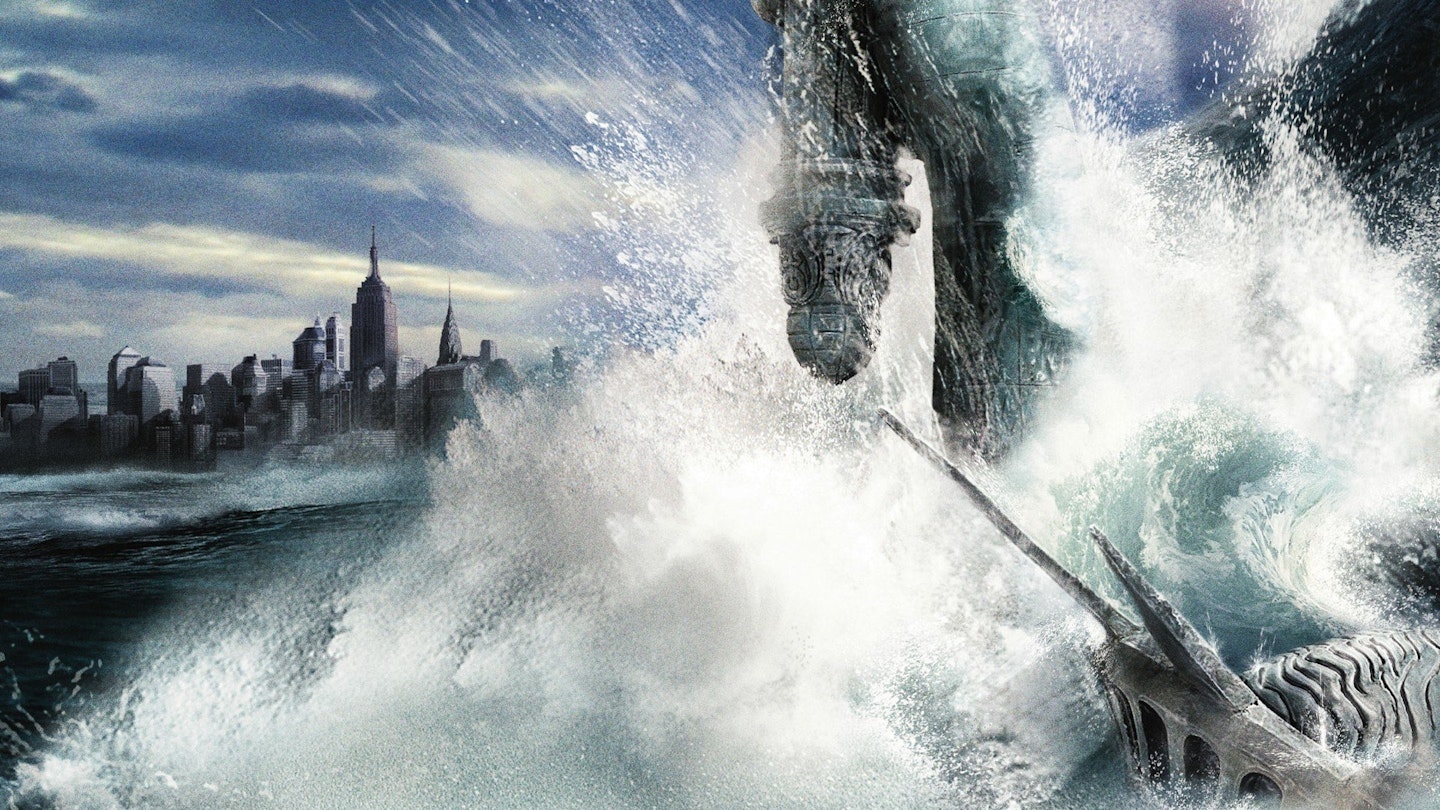A stunning, computer-generated sci-fi scene, possibly from a video game, unfolds in rich medium blues and grays. The dark, overcast blue sky looms over a silhouetted city skyline composed of various high-rise buildings, some adorned with spires. Below, a turbulent body of water, highlighted by whites and grays, features a focal point: a gigantic breaking wave. The white foam crashes dramatically against what appears to be a partially-visible statue or structure. Upon closer inspection, the right-hand side reveals the iconic crown of the Statue of Liberty, suggesting that the object in the water might be a colossal sci-fi creature advancing towards the statue. The scene merges elements of the familiar and the fantastical, creating a captivating, dystopian vista.